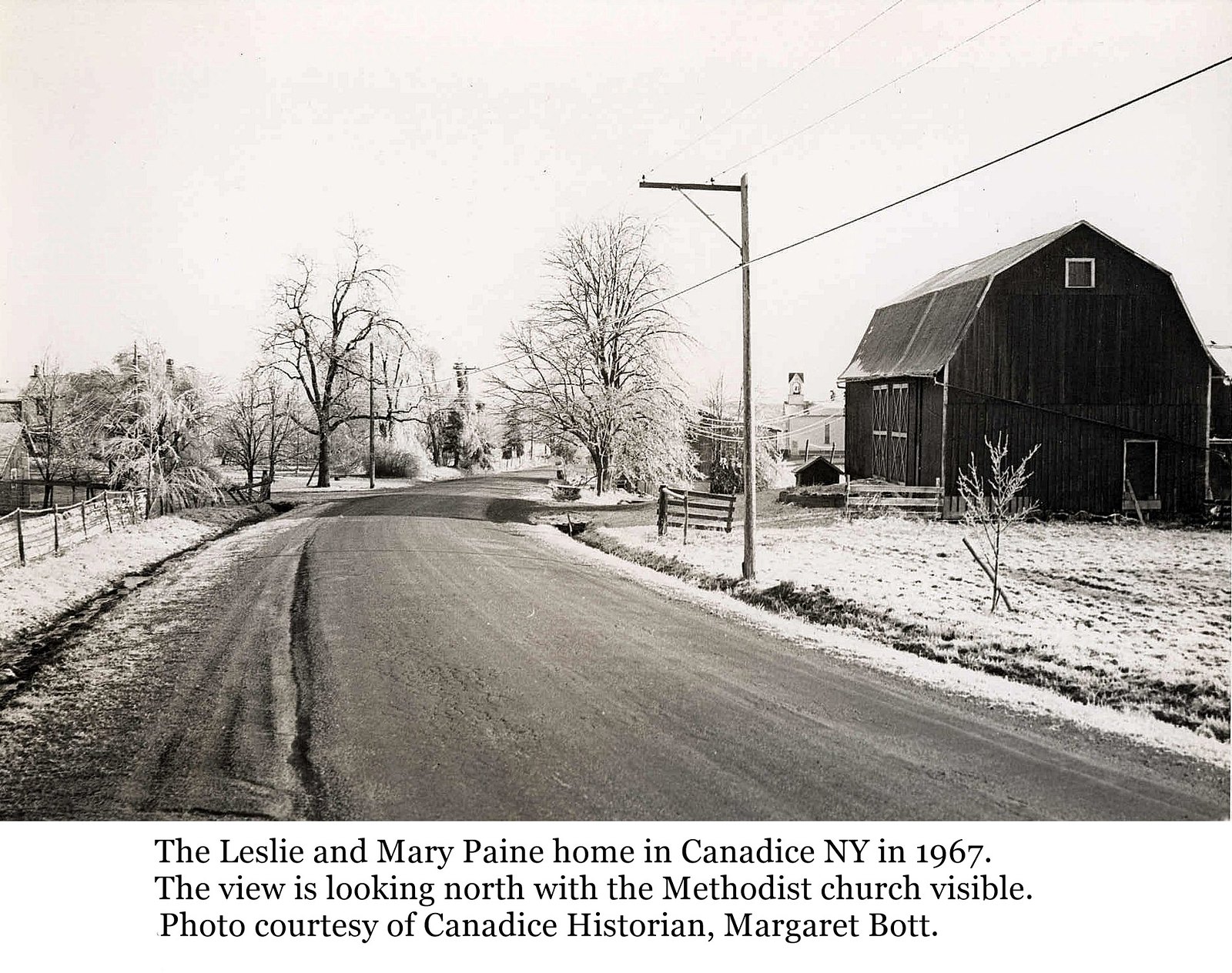In this black and white photograph from 1967, we see a snowy rural landscape in Candace, New York. A road begins at the bottom center of the image, curving to the right as it winds into the distance. The foreground features areas covered in snow on both sides of the road, with flat grassy patches visible beneath. To the right of the road, there is a large, very tall barn with vertical wooden planks and a triangle roof, topped by a window at the very peak. An electrical pole lines the right edge of the road, and a cluster of trees, dusted with snow, are situated further along the road's path. 

On the left side, behind a fence, stands another building partly obscured by trees, possibly a house. In the distance, still to the left of the road, a taller structure with a tower rises, identified as the Methodist Church. The image carries a caption at the bottom reading: "The Leslie and Mary Payne home in Candace, New York in 1967. The view is looking north with the Methodist Church visible. Photo courtesy of Candace historian Margaret Bott."